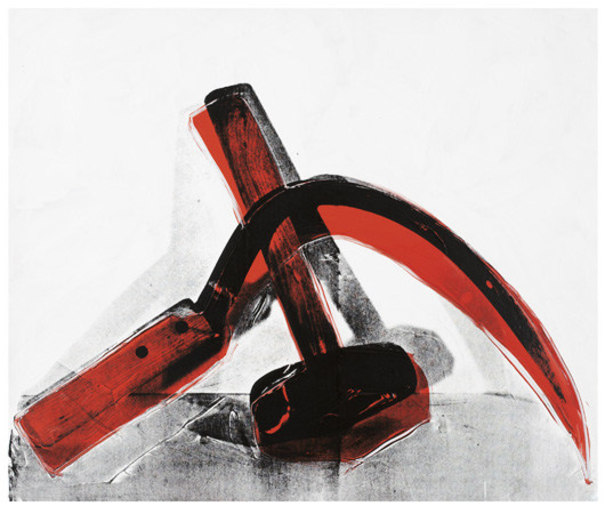This is a detailed, rectangular painting slightly wider than it is tall, featuring a rough rendering of a hammer and sickle. The background is predominantly pale grey, giving a stark contrast to the dark, charcoal-like depiction of a tabletop occupying the bottom quarter of the frame. Dominating the composition, the sickle arcs from the bottom left towards the center, pointing downwards to the right. It has a black blade outlined with a red shadow that extends to the bottom right corner. Below this element, the hammer lies with its black head resting on the table, its red-handled shaft pointing upwards to the left. The hammer is encased in a translucent red outline, casting a smudged, charcoal-like shadow on the background wall. The only color present in the painting is the vibrant red detailing on the hammer and sickle, adding significant contrast against the monochromatic setting.